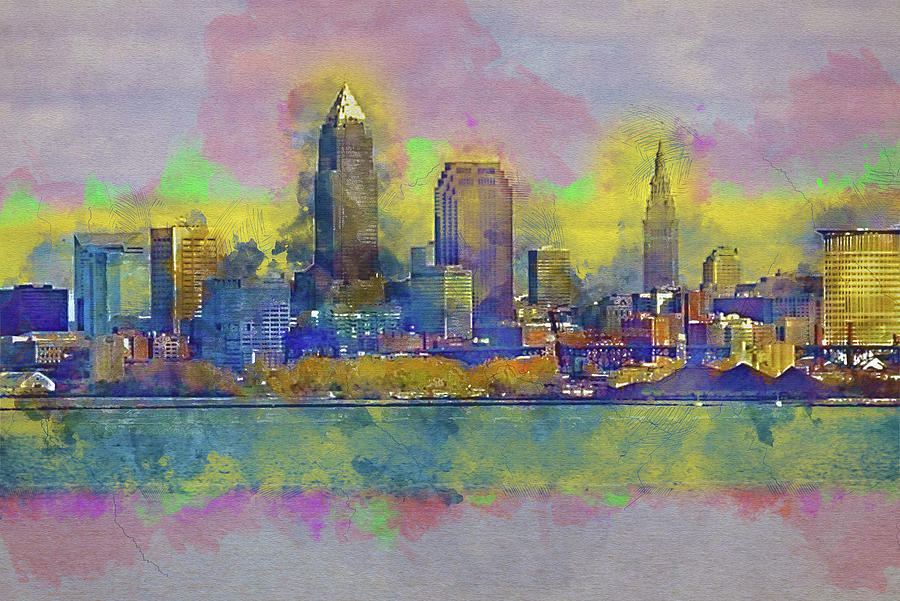This artwork portrays a detailed cityscape, possibly Chicago or New York, rendered in a computerized watercolor style with pastel hues. The city is shown from a distance across a river, with the water reflecting shades of pink, green, and blue. In the foreground, there are golden-yellowish green bushes and possibly some railroad tracks. The buildings vary in architectural styles, with the tallest one having a pointed top resembling a black square pyramid. The city's skyline is illuminated with various colors, suggesting lights in the buildings' windows. A distinctive church can be seen in the background, adding to the city's urban charm. The overall scene captures the essence of a vibrant, bustling metropolis, seamlessly blending natural and man-made elements.